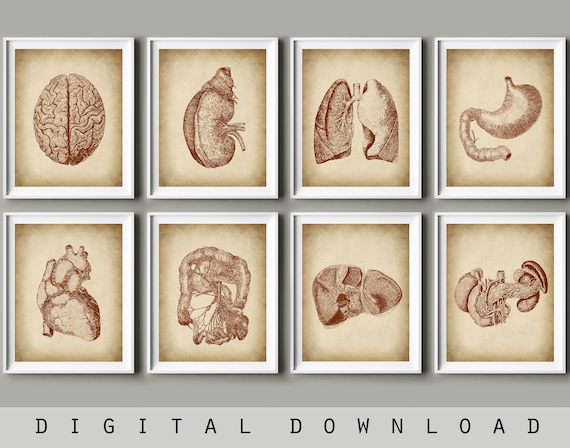This image features eight framed illustrations of human organs, each meticulously drawn in maroon ink on beige parchment paper, giving it a vintage medical textbook aesthetic. The series is arranged in two rows—four on top and four on the bottom. Starting from the top left, the illustrations include a top view of a brain, a kidney, a pair of lungs, and a stomach. The bottom row depicts a heart, a large intestine, a liver, and an unidentifiable organ. The frames are white wooden, and the background of the entire composition is a subtle dark gray. Positioned at the bottom of the image is the text "digital download" in spaced-out, black lettering on a gray strip. The detailed and realistic style of the drawings enhances the vintage feel.